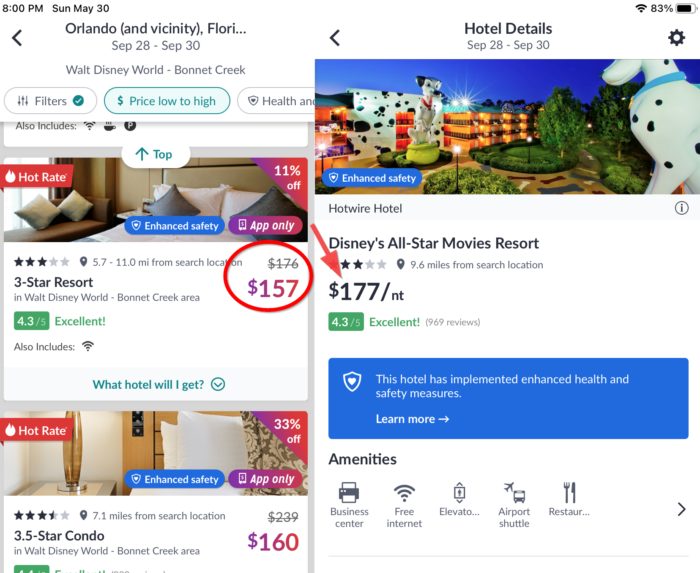This image displays a comprehensive snapshot of hotel options and pricing for the "Orlando and vicinity" area between September 28th and September 30th. Highlighted is a three-star resort in the Walt Disney World Bonnet Creek area, boasting an excellent 4.3 out of 5 rating. The listing mentions filtered prices from low to high, featuring amenities such as Wi-Fi and enhanced safety measures. The original price of $176 has been reduced to $157, with the new price circled in red to emphasize the discount. To the right, another section describes the Disney's All-Star Movies Resort, located 9.6 miles from the search location. This hotel also maintains a 4.3 out of 5 rating from 969 reviewers and similarly emphasizes its implemented health and safety protocols. Prices are marked at $177 per night, and a prominent red arrow points to this detail, ensuring visibility. In addition, a picture of two dogs amidst a cluster of trees is included, possibly indicative of pet-friendly accommodations or nearby nature attractions.